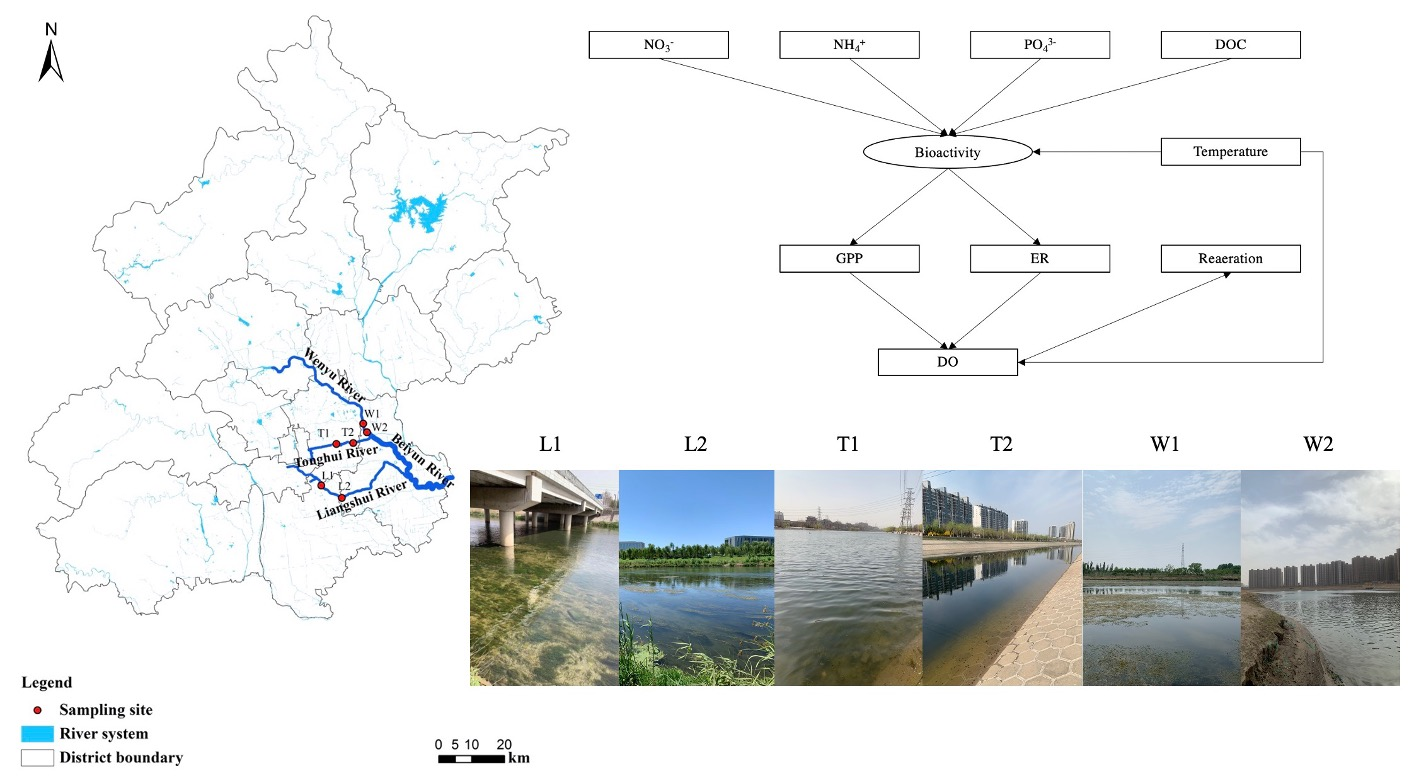The image is a detailed black-and-white map that appears to be part of an infographic centered on a river system, showing intricate details both spatially and scientifically. The map includes fine print text, making it hard to read, and features a key at the bottom indicating that blue lines represent river systems, white areas denote district boundaries, and red dots mark sampling sites. A compass at the top points north, and the region depicted seems to include the Wenyu, Belyun, Tunghu, and Lengshu Rivers, suggesting it's somewhere in Asia.

Above the map is a complex flow chart with boxes labeled by various factors involved in bioactivity, such as NO3, NH4, and PO4³. The chart also mentions parameters like temperature, GPP, ER, DO, and reaeration, although the connections between these labels are not immediately clear due to the lack of explanatory text.

Below the map are six images labeled L1, L2, T1, T2, W1, and W2, displaying actual waterways illustrating what the map references. These images help to visually correlate specific locations on the map with real-world landscapes, making it easier to understand the geographic and environmental context being presented.